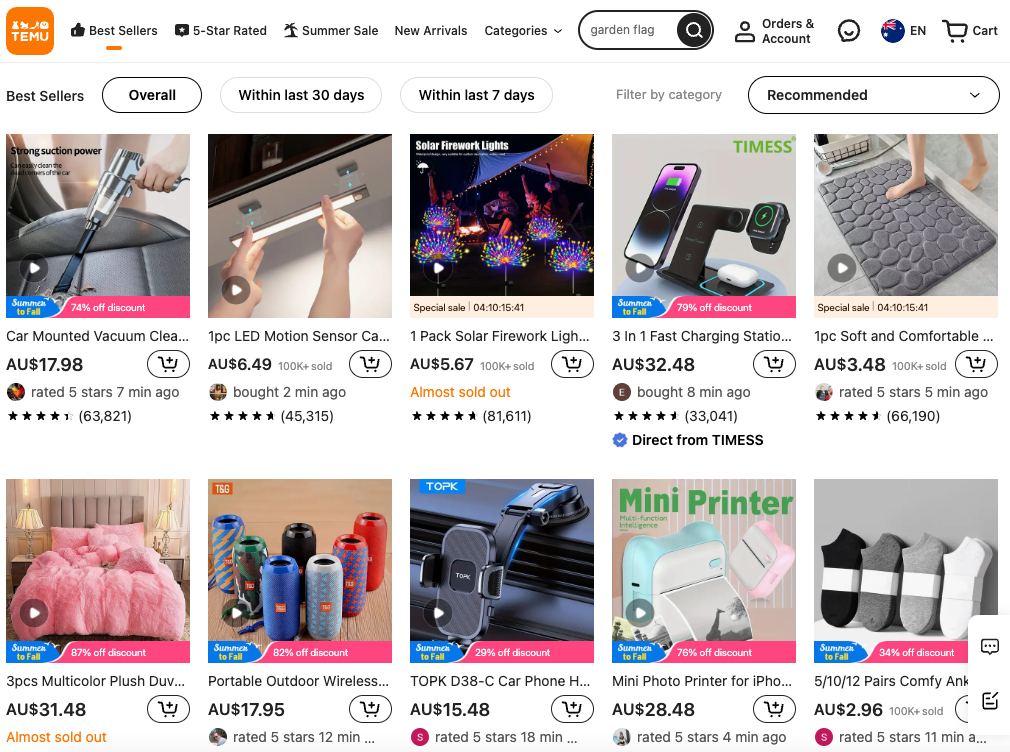The image captures a screenshot of the highly popular Chinese retail site, Timu. Positioned prominently in the top left corner is the brand's distinctive logo, situated within an orange square background. Below this, the screen showcases an extensive assortment of products available for purchase on the site. Featured items range from a car-mounted vacuum cleaner and a versatile LED strip to firework lights, a phone charging station, a soft bath mat, luxurious plush duvets, portable wireless radios, a phone mounting bracket, a compact mini printer, and an assortment of comfortable ankle socks. The diverse array caters to various needs and preferences, all offered at highly affordable prices, indicated in Australian dollars. The website's display is set to English. At the top of the page, navigation options include popular categories such as bestsellers, five-star rated items, a link to summer sale merchandise, and sections for new arrivals. Additionally, users can refine their shopping experience using the categories menu or the convenient search option located at the top of the screen.